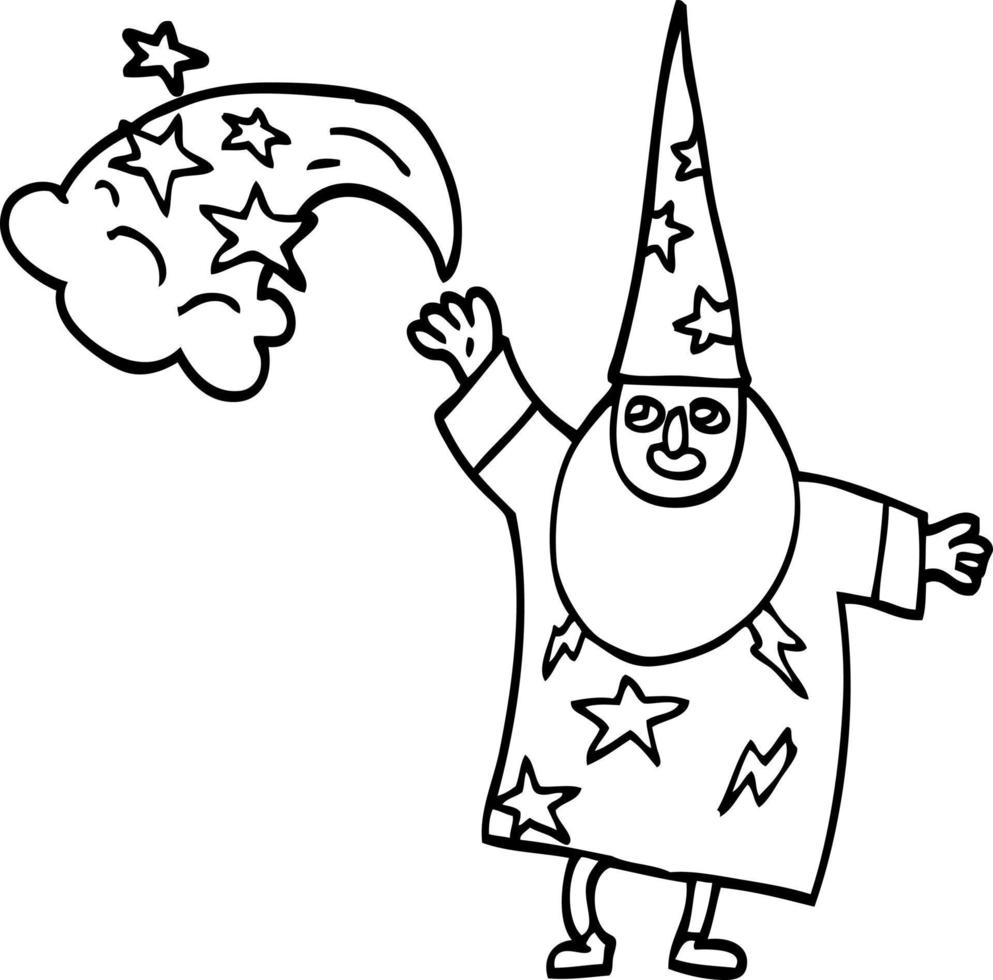The image is a detailed black and white drawing made with what appears to be a black sharpie or marker, featuring a wizard that combines a childlike simplicity with professional artistry. The wizard is depicted as a stick figure with a tall, pointed hat adorned with stars. He has a long, oval-shaped beard that stretches from ear to ear, obscuring parts of his star- and lightning-bolt-patterned robe. The wizard's spindly legs extend below his robe, and he wears pants and shoes. His left arm is raised as he casts a spell, emitting a cloud-like puff filled with stars from his hand. The wizard smiles and looks up at the magical energy. The entire image is rendered in clean, black lines on a white background, with no additional colors or shading.